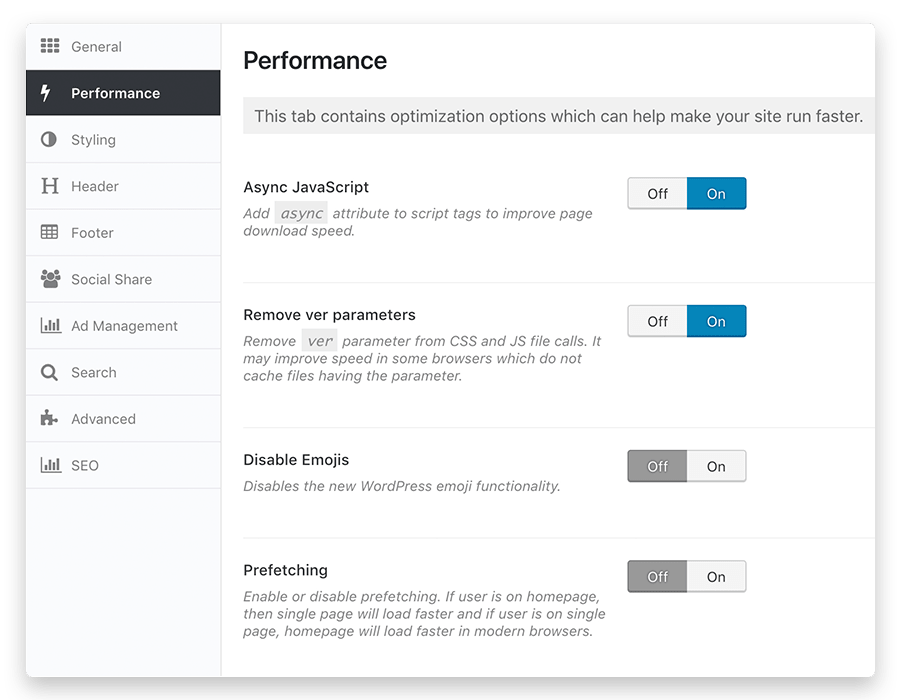This screenshot appears to be taken from a website or computer application interface focused on performance optimization settings. The majority of the interface consists of black text on a white background. 

On the left-hand side, there is a vertical column featuring various settings categories listed in a vertical stack. Each category is accompanied by a small black and white icon. The categories include: 

- **General**
- **Performance** (highlighted with white text on a black background, accompanied by a lightning bolt icon)
- **Styling**
- **Header**
- **Footer**
- **Social Share**
- **Ad Management**
- **Search**
- **Advanced**
- **SEO**

To the right of this column, the top of the screen displays the word "Performance" in black text, indicating that the Performance tab is currently active. Below this, there is a light grey rectangle extending beyond the visible edge of the screenshot, indicating that the far side of the section is cut off.

Within this Performance tab, several optimization options are displayed to help speed up the website:

1. **Async JavaScript**: Adding the `async` attribute to script tags to improve page download speed. This option has two toggle boxes, "On" and "Off," with "On" selected and highlighted in blue.
2. **Remove Query String from Static Resources**: This involves removing query string parameters from CSS and JS file calls, potentially improving speed in browsers that do not cache files with parameters. "On" is selected and highlighted in blue.
3. **Disable Emojis**: An option to disable the new WordPress emoji functionality. The "Off" option appears to be highlighted in grey.
4. **Prefetching**: This feature enables or disables prefetching to enhance page loading times. Specifically, if the user is on the homepage, the single page will load faster, and vice versa, in modern browsers. The current selection is "Off," which is highlighted in grey.

The overall design of the interface is utilitarian, focusing on providing easy access to various performance settings aimed at enhancing website speed and efficiency.